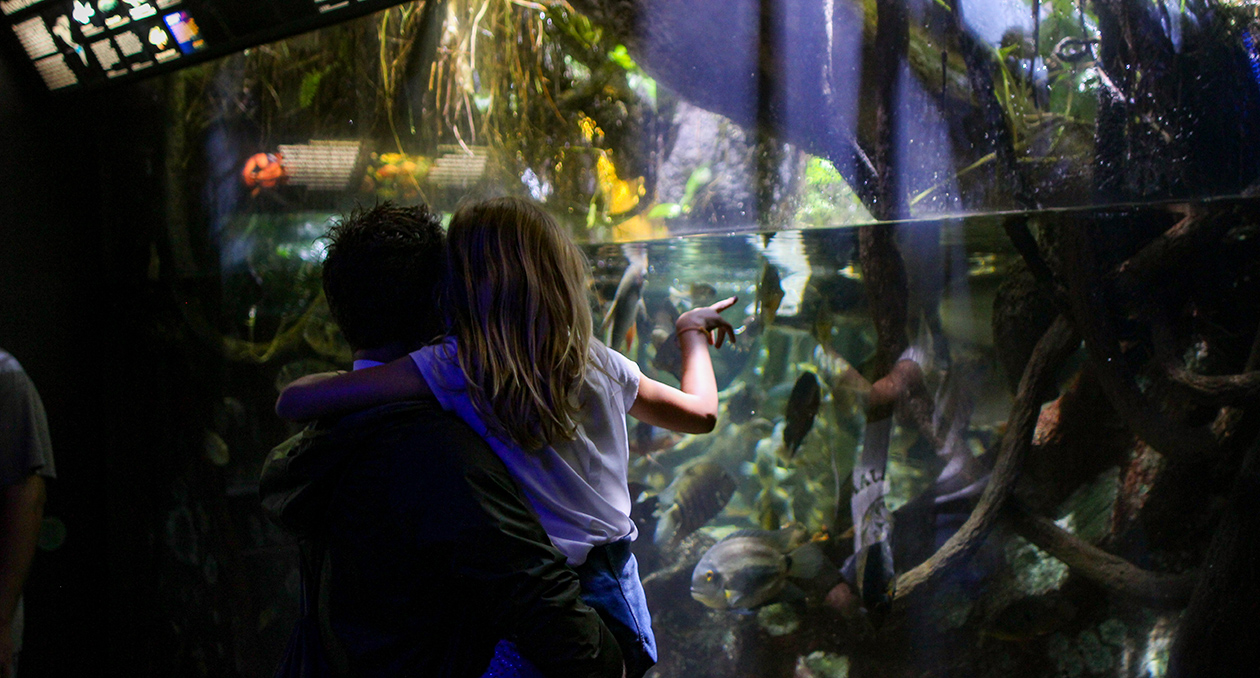In this full-color photograph taken indoors under artificial lighting at an aquarium, a man with short dark hair, wearing a green hoodie, is holding up a little blonde-haired girl dressed in a white t-shirt and jeans. They stand in front of a large glass tank filled about halfway with water, which serves as home to various fish, including angel fish and smaller species, swimming among branches and roots that suggest a tropical environment. The girl, positioned slightly left of center, points excitedly at the tank, drawing attention to the vibrant undersea life. Above the tank, a lit-up information screen is partially visible in the upper left-hand corner, casting light down onto the scene. The sides of the image are darker, emphasizing the glow from the tank and the interaction between the girl and the marine display.